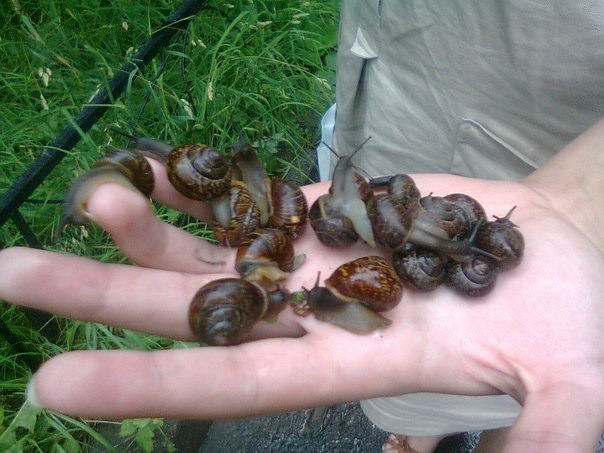In this detailed outdoor photograph, taken in landscape mode, a person's outstretched hand, palm facing up with a slight bend in the fingers and thumb oriented to the left, is covered with approximately ten to twelve snails. The person, attired in a tan-colored shirt, stands adjacent to a bright green patch of grass, hinting at where the snails may have been found. The skin of the hand appears Caucasian, with noticeable nail details, including an uncut thumbnail. The snails exhibit slimy, translucent gray bodies with some darker heads and antennae, and their shells vary from dark brown on the right to lighter brown and gray on the left. The snails' bodies appear gelatinous and wet, while their shells are clean and shiny, contributing to the intricate texture of the scene. The bottom left corner of the image might also include a hint of a foot, adding to the natural setting of the photo.